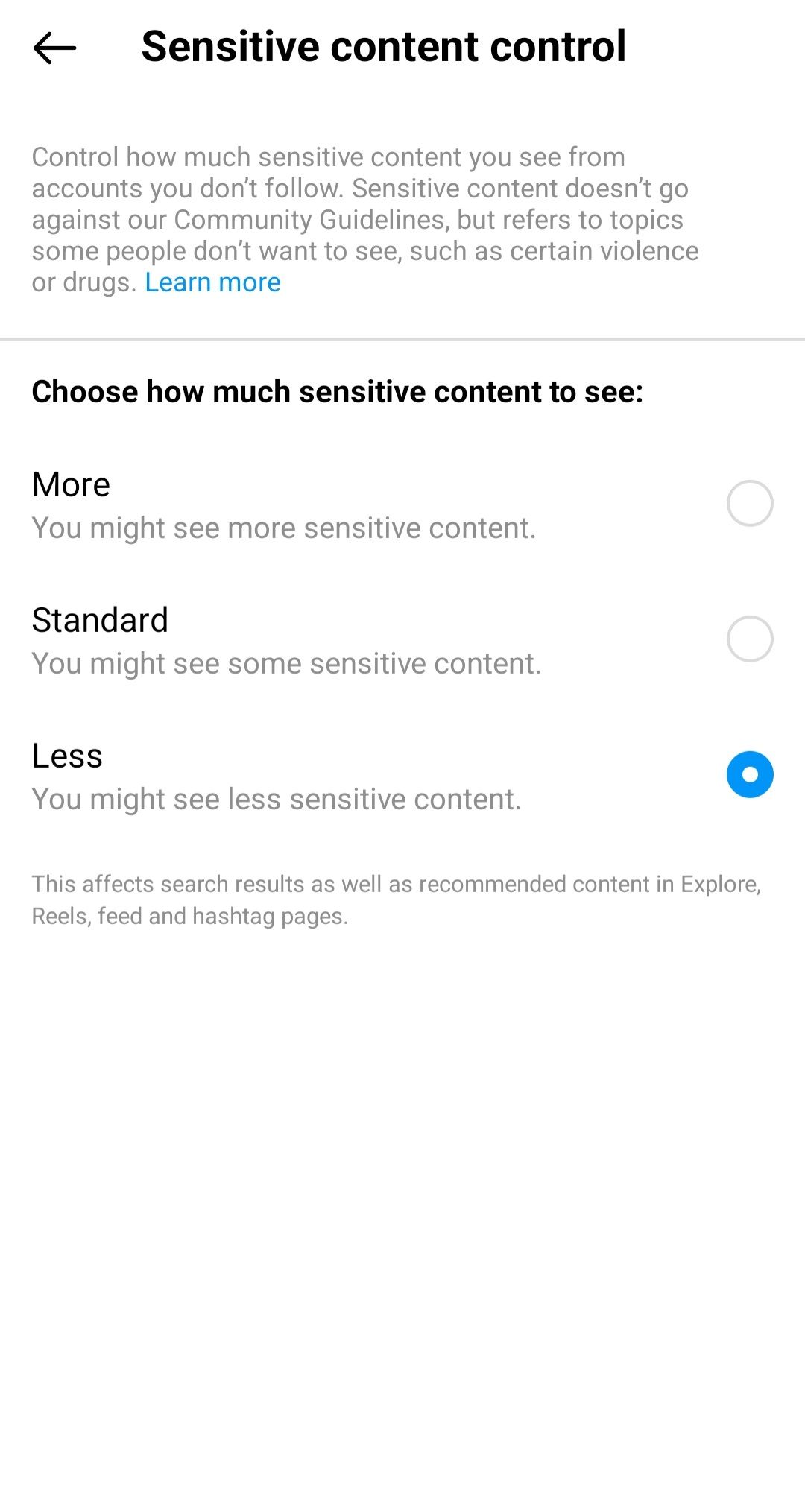In the upper left corner of the image, there is an arrow pointing to the left, indicating navigation. Next to it, in bold black text, is the heading "Sensitive Content Control". Below this heading, in smaller gray text, it reads: "Control how much sensitive content you see from accounts you don't follow. Sensitive content doesn't go against our community guidelines but refers to topics some people don't want to see, such as certain violence or drugs." 

Further down, in blue text, it says "Learn More". 

Continuing below in bold black text, the instruction "Choose how much sensitive content to see" is displayed. 

Next, three options are listed in black text:

1. **More**: Accompanied by the note "You might see more sensitive content" and an open circle to the right.
2. **Standard**: Also noted with "You might see more sensitive content" and another open circle to the right.
3. **Less**: Followed by "You might see less sensitive content" with the circle filled in blue.

At the very bottom, in light gray text, it states: "This affects search results as well as recommended content in Explore, Reels, Feed, and Hashtag pages."